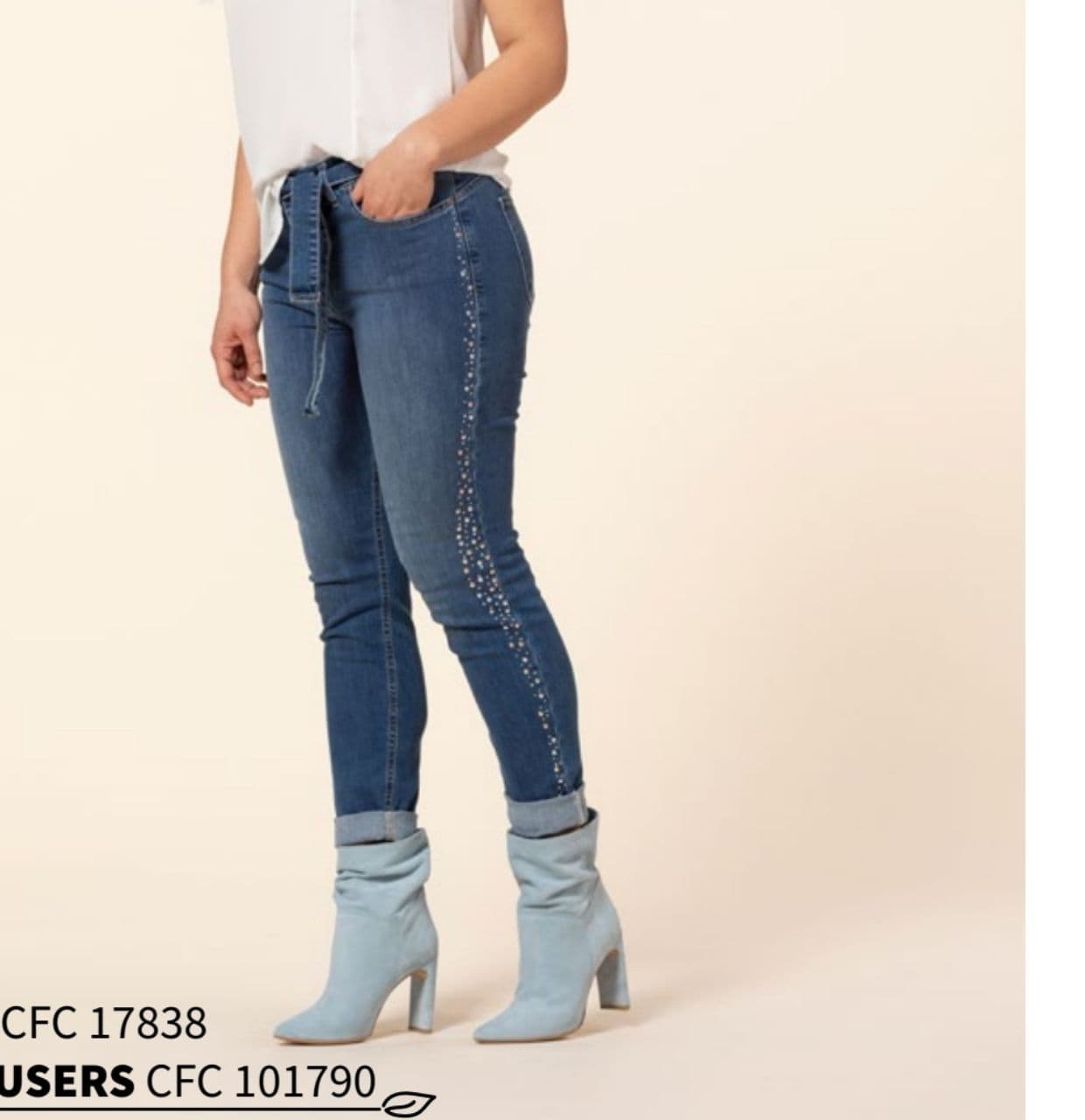The image depicts an advertisement page from a clothing catalog featuring a cropped photo of a woman, showing her body from just below the shoulders to her legs. She is dressed in a white, somewhat baggy blouse with her bare arms visible. She pairs this with tight, faded blue jeans adorned with rhinestones along the outer leg seams. Around her waist is a tie belt made from matching denim material. Her jeans are rolled up at the cuffs, which reach the tops of her light blue, short boots that have 3-inch heels and rise two inches above the ankle. The background of the image is light-colored with subtle shading. In the bottom left corner, the text "CFC 17838" is visible in capital letters, and underneath it, also in bold capitals, is the word "USERS" followed by "CFC 101790."